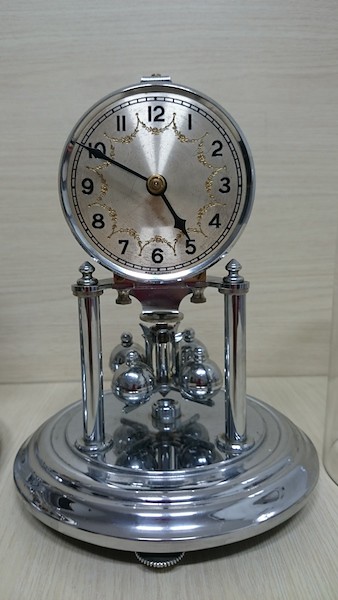This image features an antique-style mantel clock, reminiscent of classic home decor. The clock boasts a polished silver exterior accented with elegant gold highlights on its face. It stands on a refined silver platform, supported by two pillars that frame its intricate design. At the heart of the clock, four ornamental balls reside, likely designed to oscillate rhythmically like a pendulum, enhancing its vintage charm. The clock face prominently displays clear Arabic numerals, making it easy to read, flanked by sleek black hour and minute hands. The hands are connected at a central brass-colored knob, adding a touch of sophistication to the overall aesthetic. This captivating timepiece combines practicality with timeless elegance, making it a striking addition to any mantel.